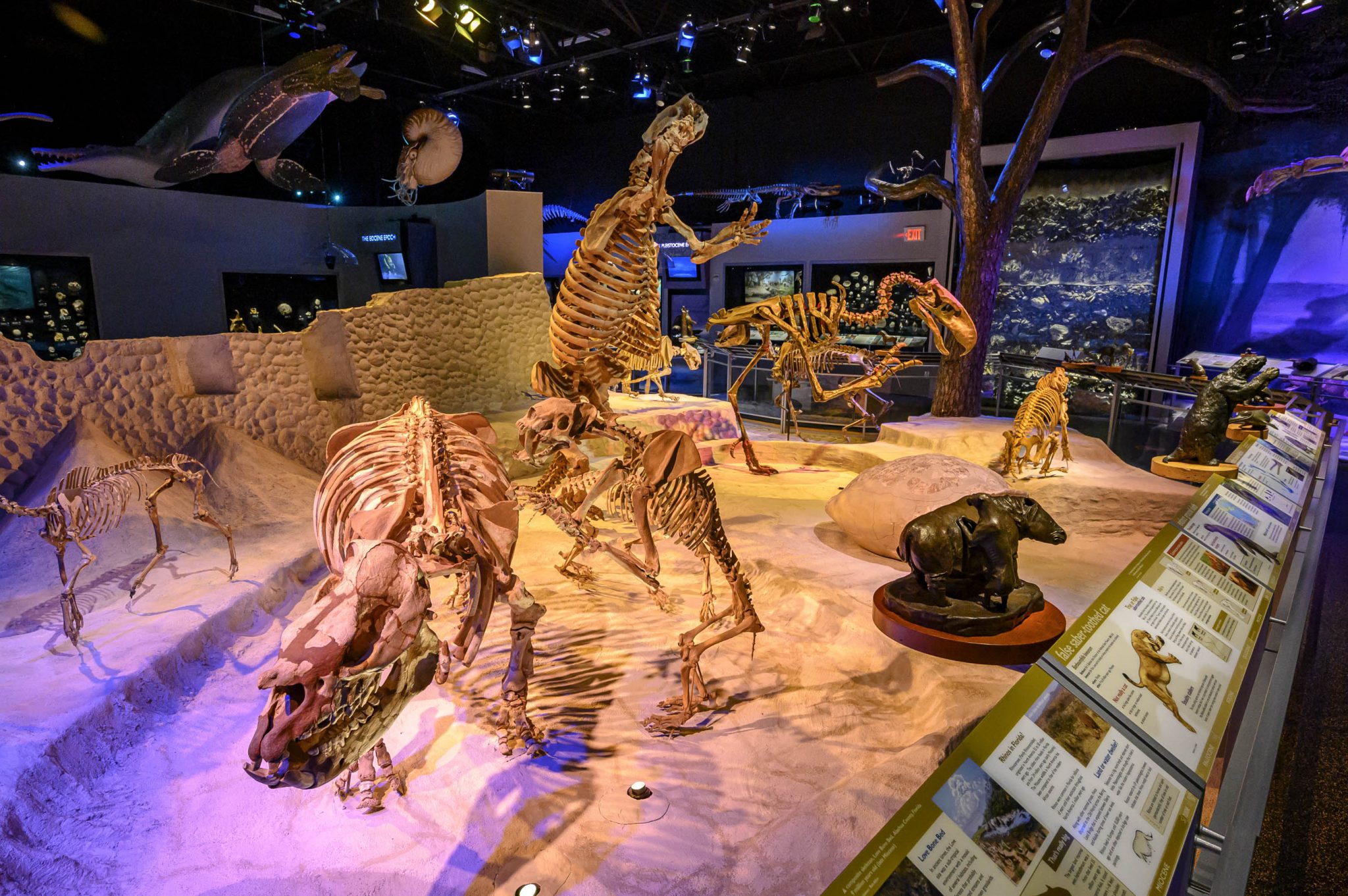The photograph is set indoors within a museum, lit by artificial lighting. It appears to be a square, full-color image without a definitive border or specific background. The primary focus is on a detailed diorama featuring prehistoric skeletal models poised on a large, flat table with a tan, sand-like surface. The table holds at least five to six skeletons, primarily of mammals, as indicated by their structural features. 

Foreground includes a quadrupedal skeletal predator with a long, craned neck and an oval-shaped head, while behind it stands a larger bipedal skeleton with a broad, oval body, long slender neck, and a distinctive skull, appearing to resemble a dinosaur. A recognizable T. rex model is also present, distinguished by its large hind legs, middling body size, small forearms, and large head with wide jaws. Surrounding the table are informational white pages with photographs, diagrams, and descriptive text.

The background of the image features a high, black ceiling illuminated by colored lights, enhancing the various display units within the museum. Along the back wall, gray and adjacent to the table, are four metal-framed computer kiosks designed for interactive displays, and possibly additional exhibit panels that might include marine creatures. The lighting in the room incorporates darker tones, including black lighting, creating a vivid yet subdued atmosphere ideal for highlighting the prehistoric displays.